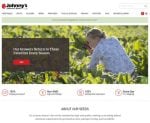The image is a highly blurry screenshot of a website's front page. In the upper left corner, a red logo is visible, accompanied by black text that seems to spell out "Johnny's." The adjacent text is indecipherable due to the image's blurriness. A breadcrumb menu is faintly perceptible beneath the logo.

Dominating the central area of the page is a large photograph of a green field, featuring a woman bent over, tending to the crops or plants. Superimposed on this image, on the left side, is a black box with white text, though the blurriness makes the text unreadable. Below this black box, there is a red call-to-action button, also rendered illegible by the image quality.

Further down the page, there are four indistinct sections of text spread horizontally across the screen, their contents obscured by the blur. Centrally aligned beneath these sections is another unclear text block, adding to the overall indiscernibility of the screenshot.